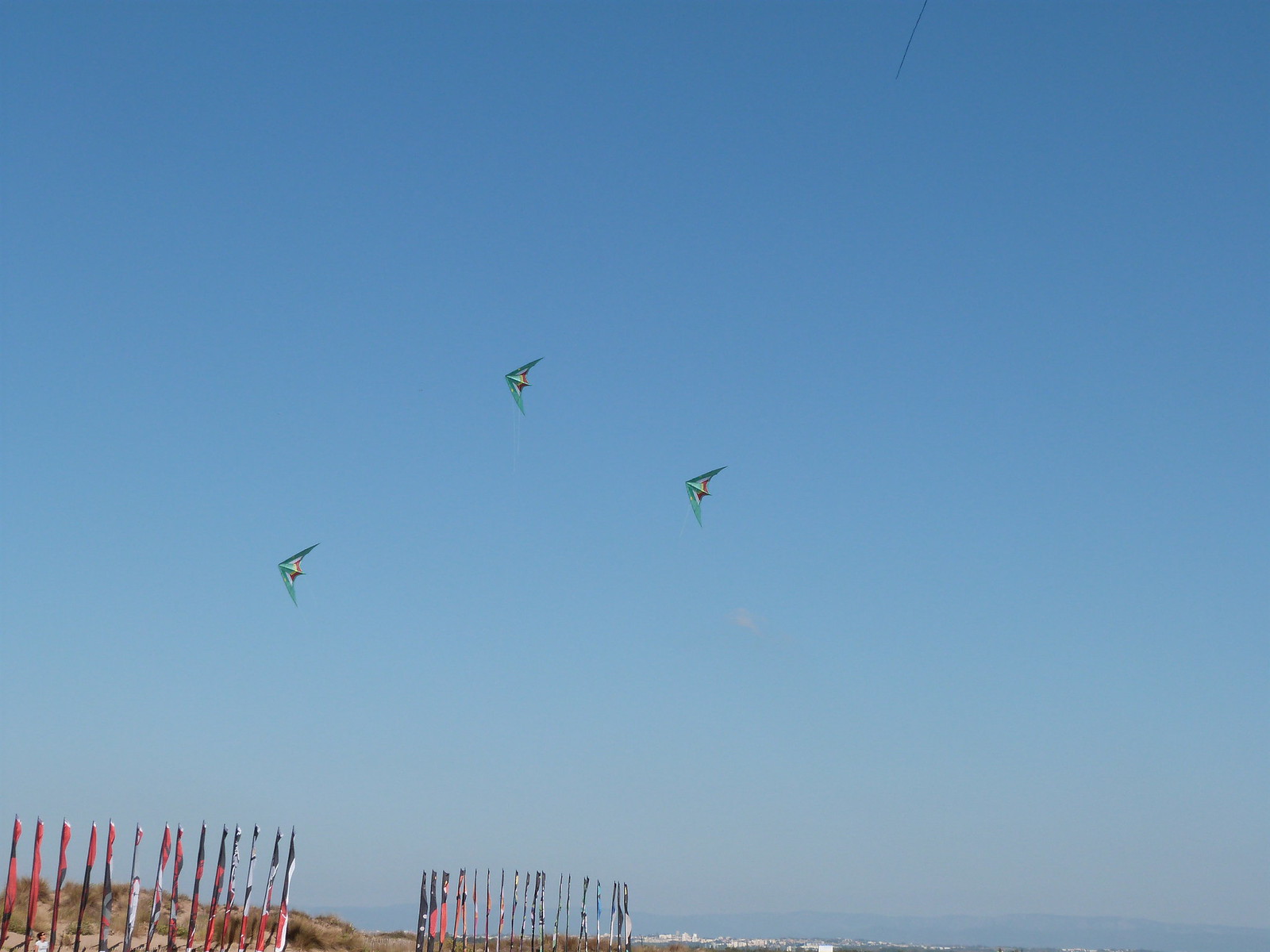In this vibrant photograph, three identical kites dominate the clear blue sky, their pointy forms and angular design giving them an illusion of sleek stealth fighters as viewed from below. Each kite features green wings, a white center body, and a red tail section. They are flying perpendicular to the ground, seemingly driven by a strong wind. The setting appears to be a beach, with the faint outline of a sandy dune visible in the bottom left corner. Below the kites, in the lower left of the frame, there are rows of flag poles, each wrapped with furled flags in red, blue, and white. Further in the distance, one can discern the outline of white dwellings and a mountainous ridge, all set against the expansive crystal blue sky. The photograph captures a moment of dynamic stillness, where the kites soar and the world below quietly unfurls.